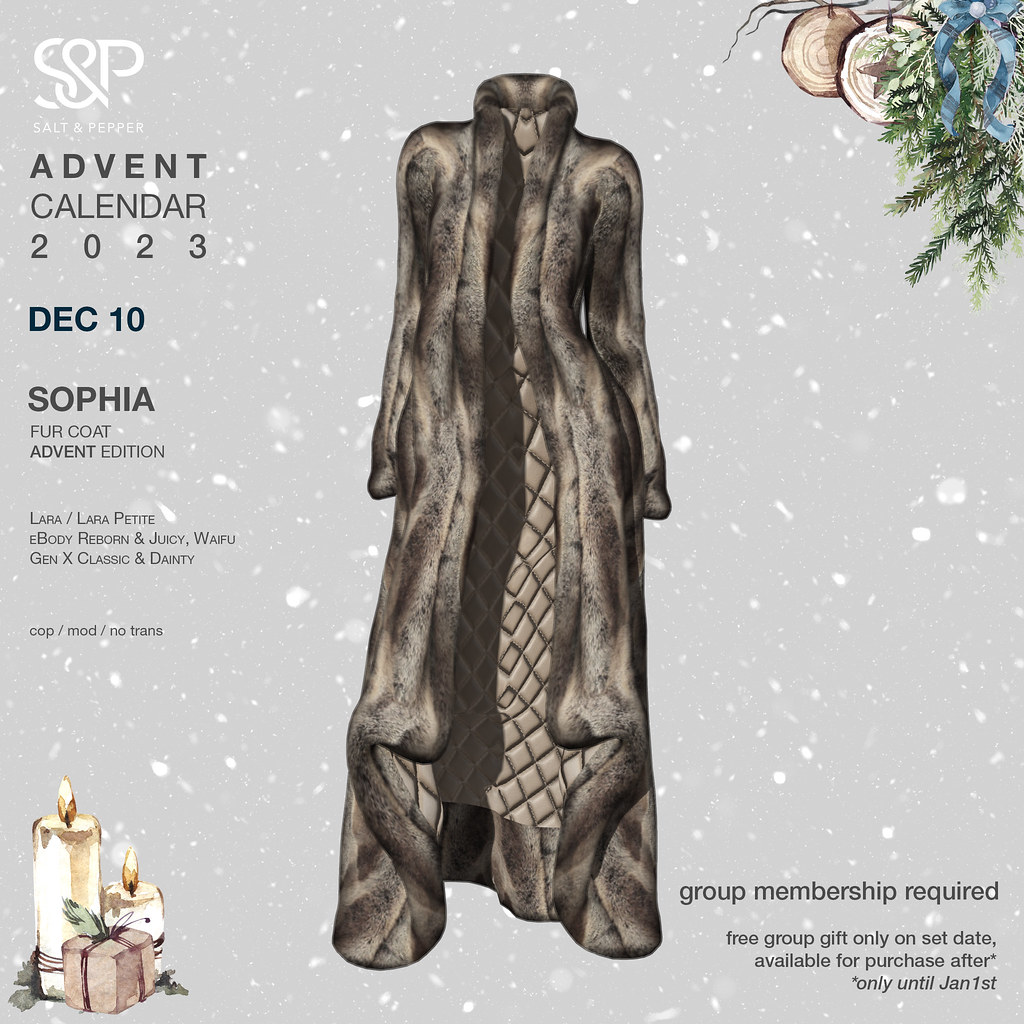This image is an advertisement for the Salt & Pepper (S&P) Advent Calendar 2023. The background showcases a light gray color with white spots reminiscent of snow. Centrally, a long, mottled light brown and black fur coat is prominently displayed. In the top left corner in white text, it reads "S&P," followed by "Salt & Pepper" in black text, with "Advent Calendar 2023" beneath it. Further down, it specifies "December 10," then "Sophia Fur Coat Advent Edition," and details the compatible body types: "Laura, Laura Petite, eBody, Reborn, Juicy, Waifu, Gen X, Classic, and Dainty." It also notes "Cop, Mod, No Trans."

The bottom left corner features an old-timey drawing of two candles and a present with a pinkish coloration. In the top right corner, a depiction of a pine tree branch adorned with a blue ribbon and two ornaments can be seen, adding to the festive theme. The bottom right corner states "Group Membership Required. Free group gift only on set date. Available for purchase after* *only until January 1st."